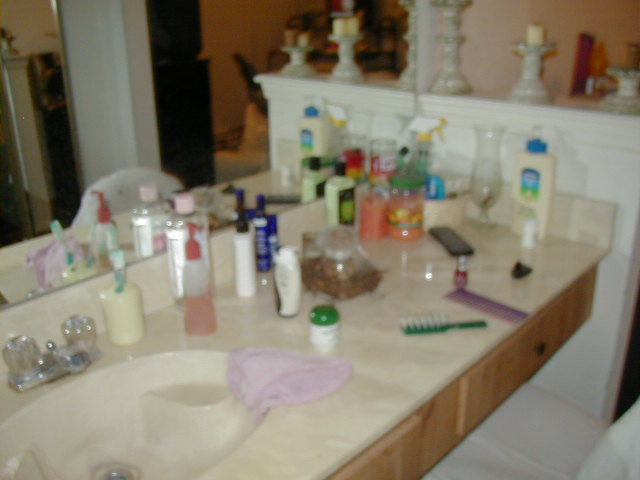In this slightly blurry photograph, a detailed view of a bathroom vanity is captured. The vanity features white-blonde wood drawers adorned with sleek black pole handles. The creamy-colored sink top is complemented by glass knob-style sink handles and a silver faucet. A white partition with a small ledge runs along the back of the countertop, topped with candles in white holders.

The items on the bathroom sink include a white, blue, and green bottle of lotion, a green comb or brush, and a purple comb. A pink bottle of hand soap, a white toothbrush holder with a green toothbrush, and a purply washcloth draped over the sink also adorn the vanity. 

Above the sink, a mirror reflects the scene, while additional items clutter the countertop. These include a clear bottle with a pink lid, a green bottle with a dark lid and green label, a spray bottle with a white lid and yellow accents, and a bottle of burgundy-colored nail polish nestled behind the purple comb and a black object.